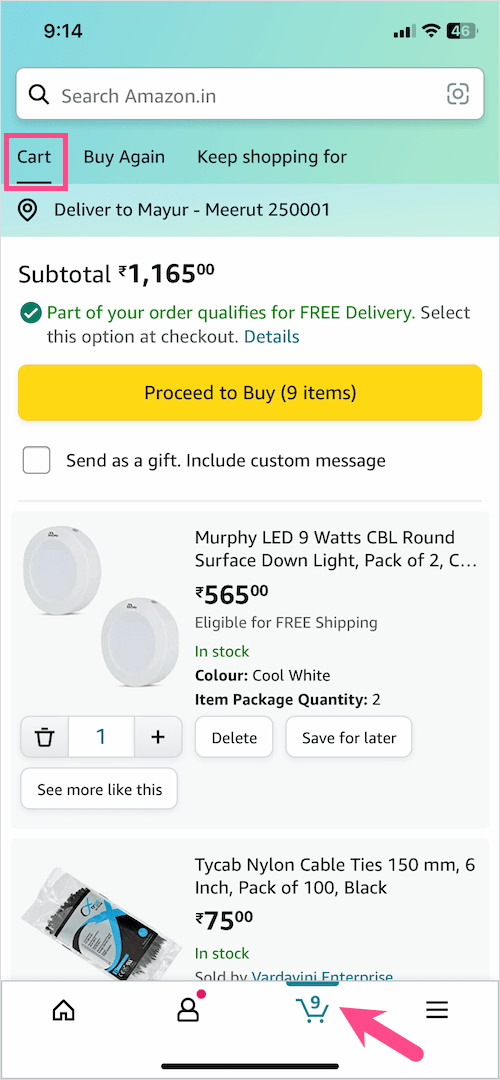This screenshot depicts the Amazon.in mobile app interface. At the very top, there's a search bar featuring a magnifying glass icon on the left. Within this interface, a pink square highlights the shopping cart icon, revealing a subtotal of ₹1,165. The delivery destination is specified as "Mayor Meerut 250001." Below this, a prominent yellow button with bold black text prompts the user to "Proceed to Buy (9 items)". Additionally, a checkbox option titled "Send as a gift" remains unchecked.

Displayed items in the cart include the "Murphy LED 9 Watts CBL Round Surface Downlight (Pack of 2)" – visually represented by an image of two white, circular plastic lights. Beneath this, the next listed item is "Cable Ties".